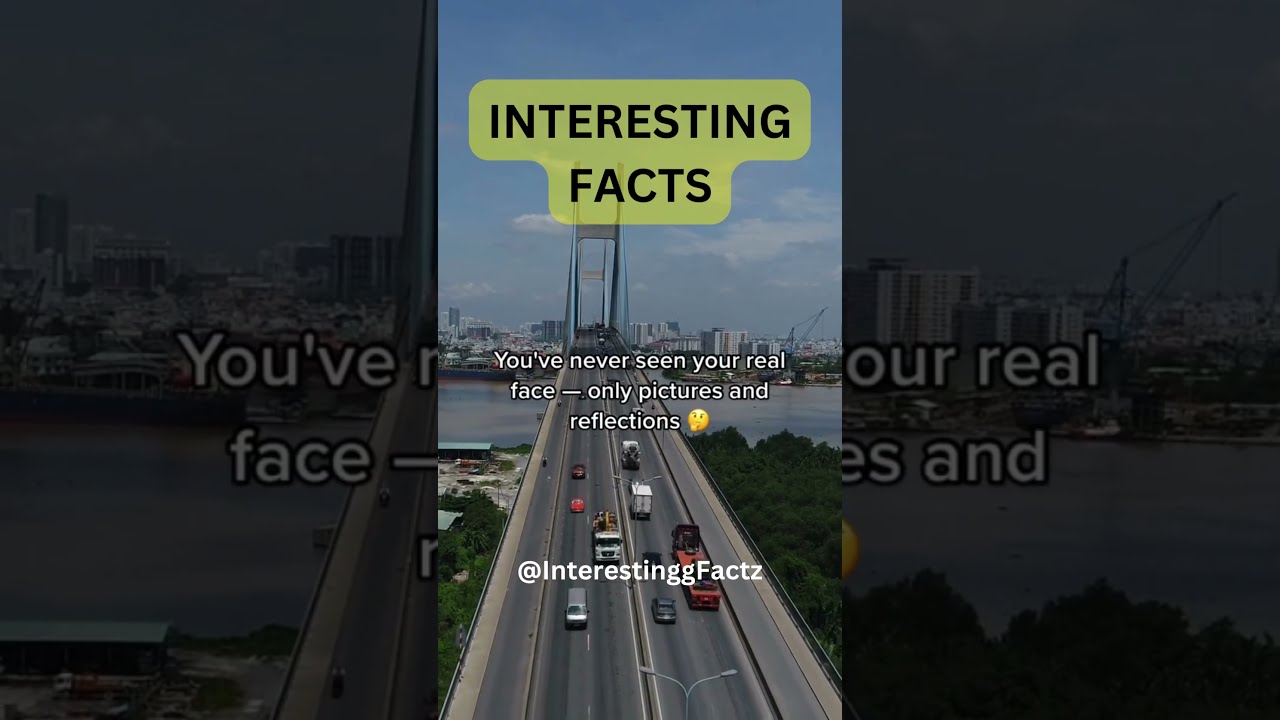This is a screenshot from a social media video, perhaps a YouTube Short or a TikTok, labeled "interesting facts" in the largest and most prominent black Arial font over a yellow overlay at the very top. Below it, in slightly smaller text, it reads, "you've never seen your real face - only pictures and reflections," accompanied by a thinking emoji. The handle of the channel, appearing at the bottom, is displayed as "Interestinggfactc". The background features a detailed cityscape with a blue, steel-beamed bridge extending over a river. The bridge supports a busy four-lane, two-way highway, with three lanes in each direction filled with various cars. The scene is set during daytime with a blue sky dotted with clouds. In the distant horizon, the outline of city buildings is visible, along with greenery in the foreground. Additionally, a big yellow smiley face is positioned near the shoreline to the right of the bridge.